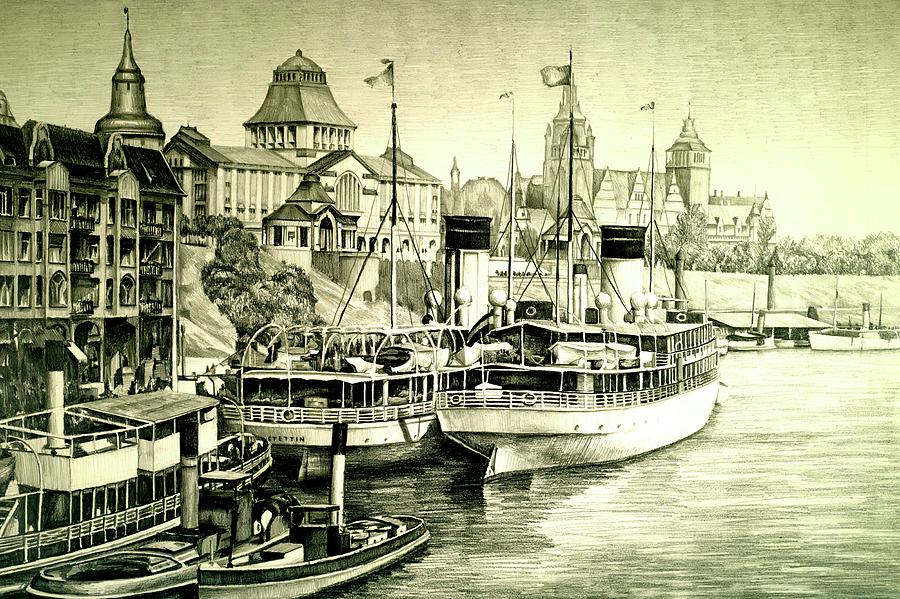This image is a detailed hand-drawn pencil illustration, predominantly in black and grey tones, depicting a historical European coastal town, possibly from the 19th century. The setting features a bustling harbor with several steamships and boats, including passenger vessels with multiple decks, flagpoles, and smokestacks, central to the composition. In the foreground, there are a couple of small shallow steamships, one of which bears the text "Stetton" on its stern. The harbor appears to be an inlet or dock area for loading people or goods. Rising above the waterfront, the left side of the illustration showcases old, multi-story buildings with intricate architectural details, and trees scattered in the background. The meticulousness of the drawing captures the essence and beauty of this historical scene, bringing life to the ships, boats, and urban landscape.